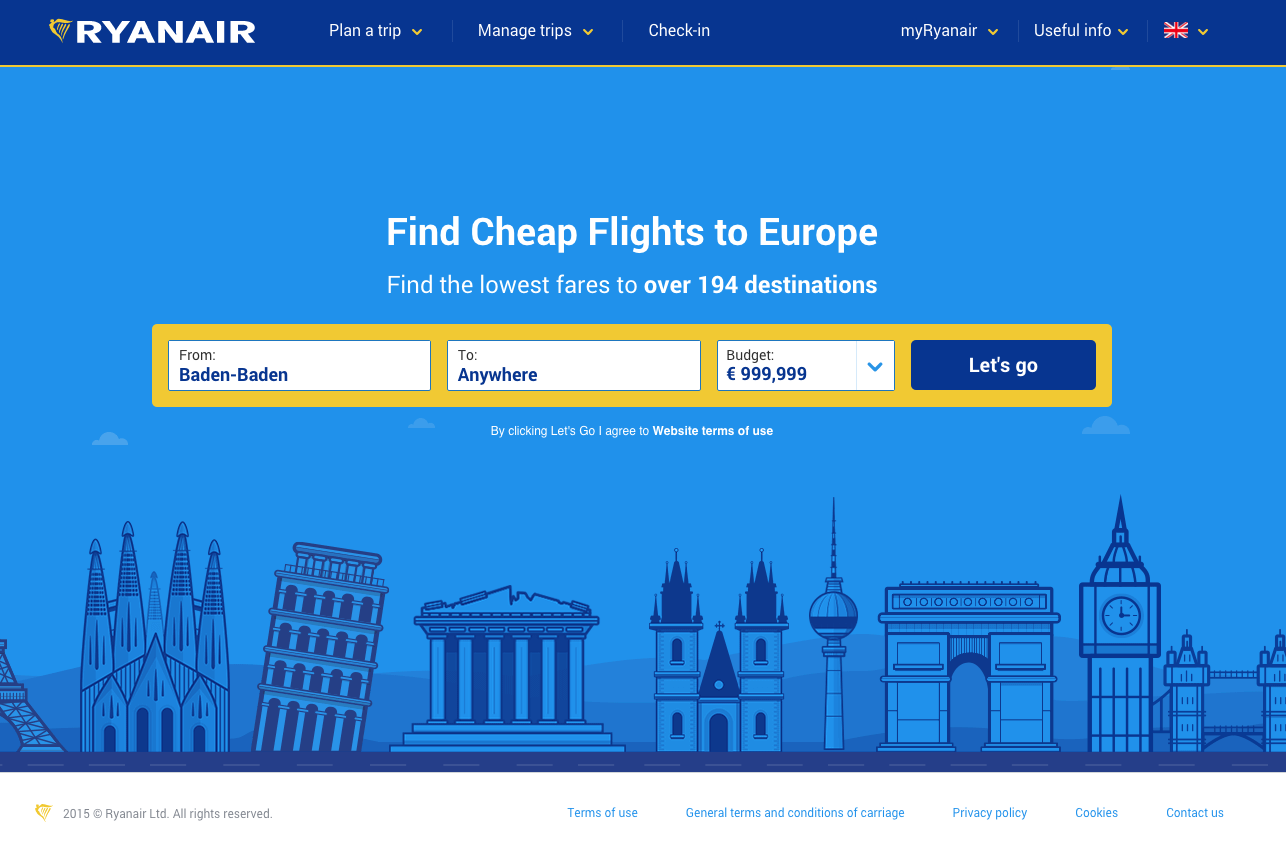This screenshot captures the homepage of the Ryanair website. In the top-left corner, the Ryanair logo is prominently displayed, featuring the company name in bold letters accompanied by a small yellow graphic element. The website’s background is a soothing light blue, which complements the detailed illustration of an ancient cityscape at the bottom. This scenic artwork includes prominent landmarks such as Big Ben, the Eiffel Tower, the Space Needle, the Leaning Tower of Pisa, and the Roman Colosseum. There's also a significant large cathedral and a bridge reminiscent of those found in London.

In the center of the website, a bold heading reads "Find Cheap Flights to Europe." Below this, the search form displays the input criteria: flights from Baden-Baden to any destination, with a budget set at 999 Euros.